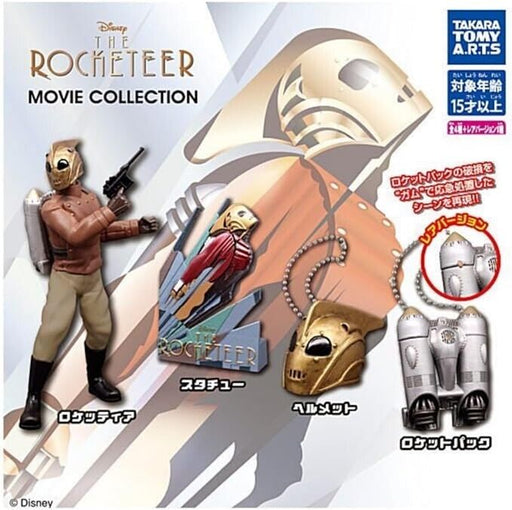This composite image showcases the Rocketeer movie collection prominently featuring Disney's The Rocketeer in gold and black text. The background is grayish-white, and a blue label on the top right reads "Takara Tomy Arts." Below this label, there's Japanese (or possibly Chinese) kanji script. The image also displays several figures and accessories related to the Rocketeer character. 

In the foreground, there is a detailed action figure of the Rocketeer, marked by his signature golden helmet with large eye caps, a silver jetpack, brown leather pants, and dark black boots. He holds a handgun in his right hand. Another figure shows the Rocketeer in a dynamic flying pose, donned in a brown leather jacket, beige pants, and black boots. Additional items include a standalone figurine of the Rocketeer helmet, a separate figurine of the jetpack, and these last two accessories appear to be keychains. Despite the language barrier with the accompanying text in Japanese kanji under each figure, the image collectively celebrates the iconic elements from the Rocketeer movie, exemplifying its memorabilia and detailed collectibles.